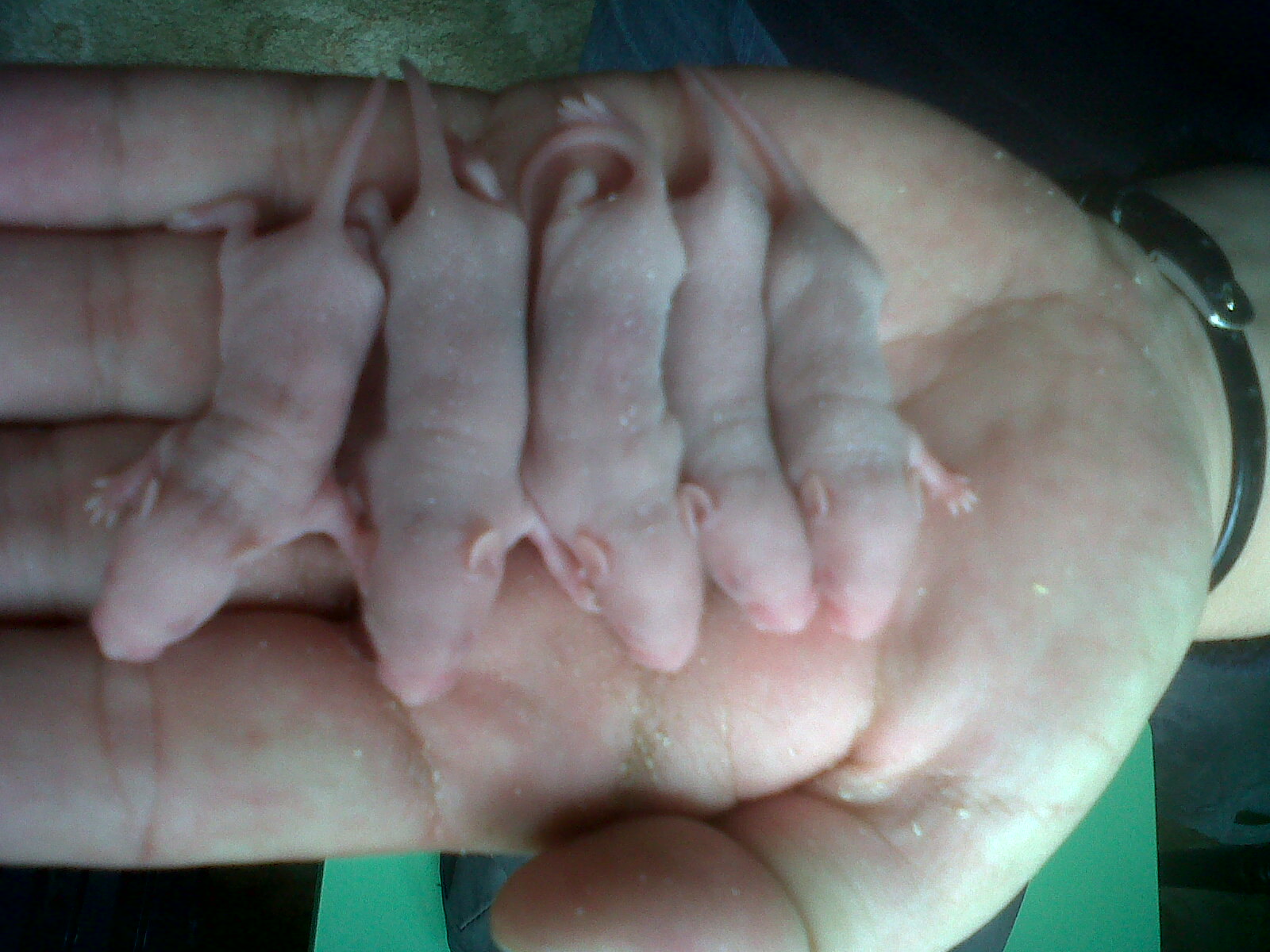In the image, we see an extremely close-up view of a Caucasian person's left hand, palm up, cradling five tiny, newborn baby mice. The baby mice are completely hairless, light pink in color, with their eyes closed and delicate feet visible. Their tiny pink tails drape over the person's fingers and the edge of their palm. The mice are so small, they fit comfortably in the palm, showcasing their fragile and freshly born state. The person holding them wears a black wristwatch with a metal strap. In the background, there is a green pattern along with black areas visible in the bottom left and top right corners, adding contrast to the scene. The hand appears to have some calluses or dry skin, adding texture to the close-up shot.